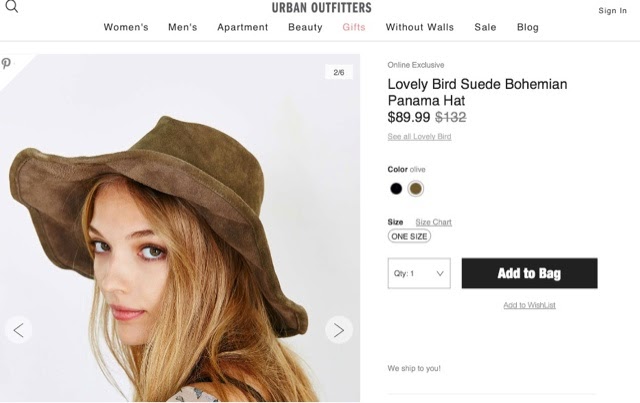The image displays the online retail site, Urban Outfitters. In the top left corner, there's a search bar, while the top right features a sign-in option. Directly below the main Urban Outfitters logo, there's a navigation menu with sub-sections including Women's, Men's, Apartment, Beauty, Gifts, Without Walls, Sale, and Blog.

At the center of the screen, an advertisement catches the eye: a young woman wearing a bohemian Panama hat made from suede. The text next to her reads "Online Exclusive: Lovely Bird Suede Bohemian Panama Hat," indicating a special deal. Originally priced at $132, the hat is now on sale for $89.99. The hat is available in two colors, black and brown, with the image showcasing the brown version. The product comes in one size only, but a size chart is accessible for detailed measurements. Shoppers can specify the quantity and add the hat to their shopping bag using a button featuring white text on a black background.